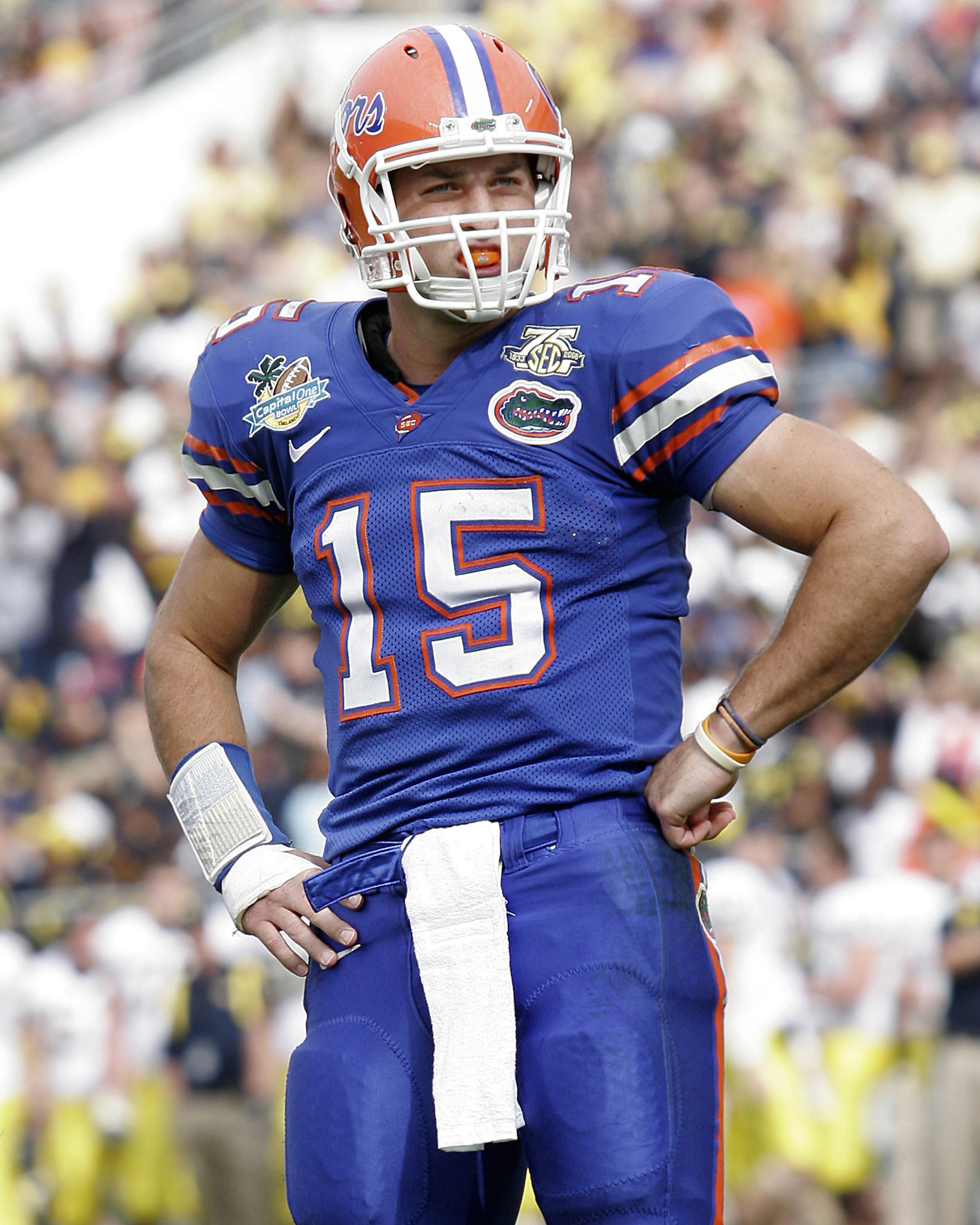In the photograph, the football player stands prominently from the knees to the top of his head, exuding the poised stance of an athlete on the sideline. His uniform is a striking combination of blue and orange, with blue form-fitting pants adorned with noticeable orange stripes down the sides. The padding underneath the pants is outlined clearly around his upper thighs. A blue fabric belt rests at his waist, from which a white towel dangles in front.

His blue jersey features the number 15 boldly displayed on his chest in large white numbers framed with an orange border. The shoulders of the jersey are padded, adding to his imposing figure. The sleeves show an alternating pattern of white and orange stripes, echoing the team's vibrant color scheme. His orange helmet, marked by a blue and white stripe down the middle, conceals a visor and an orange mouthpiece, which he is currently wearing. Above the number on his chest, a small gator logo is visible on the top right of his jersey.

Additionally, his arms are bent with his hands resting on his hips in a casual, perhaps contemplative posture. His right wrist sports a wrist guard and possibly a glove, hinting at a prior injury, while rubber bracelets adorn his left wrist. In the background, albeit out of focus, a crowd of spectators in the stands adds a vibrant yellow hue to the scene, emphasizing the lively atmosphere of the game.